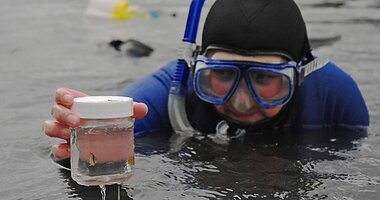A snorkeler, dressed in a long-sleeved blue wetsuit and a black hood, emerges from a body of water, likely a lake or river, which has a few visible pieces of trash. The snorkeler is laying on their stomach with their cheeks appearing flushed beneath large, blue scuba diving goggles. They are equipped with a snorkel that has a clear mouthpiece and a blue section attached to the mask. In their hand, they hold a clear jar filled with water, sealed with a white screw-top cap, suggesting they might be collecting water samples. The scene captures a blend of environmental observation and recreational diving.